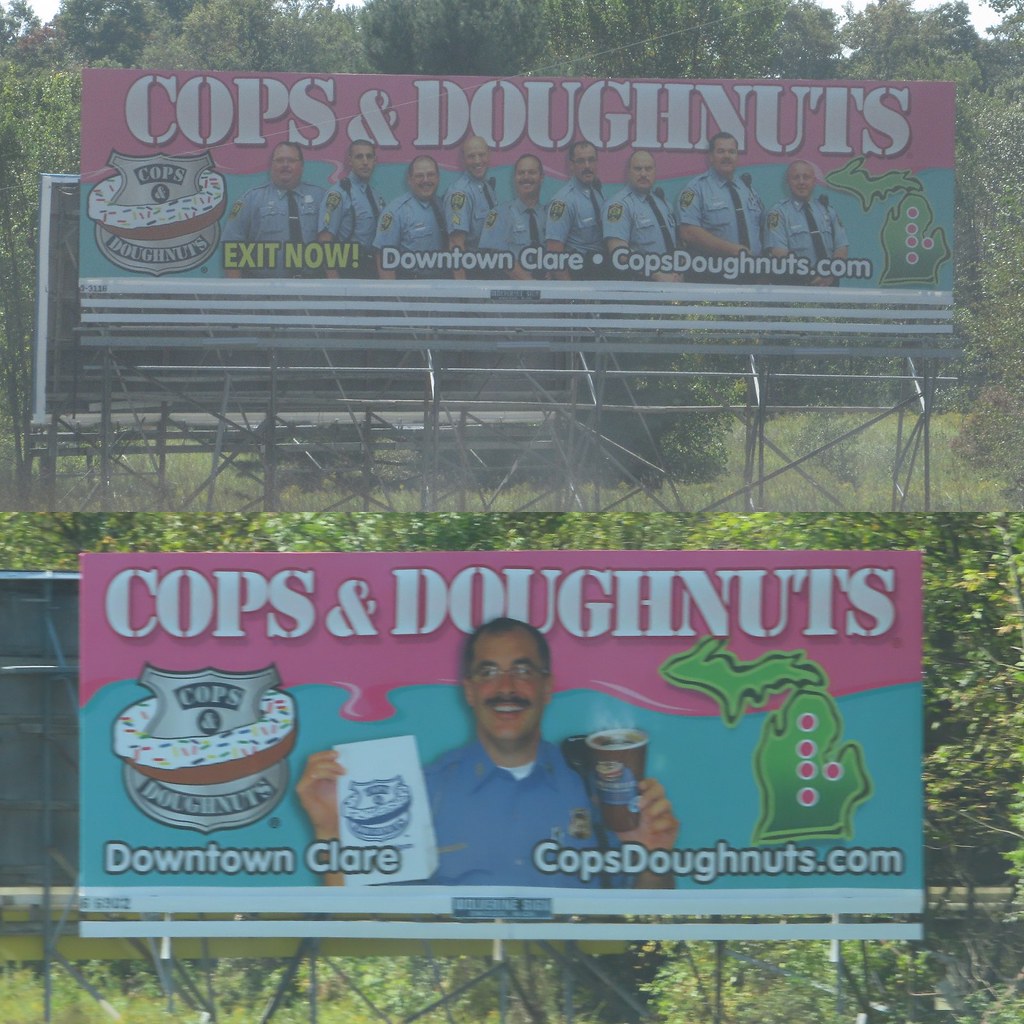This image features a promotional billboard for "Cops & Doughnuts," a bakery located in downtown Clare. The main billboard showcases a group of nine police officers, all male and seemingly Caucasian, lined up and smiling at the camera. Above them, a large badge logo reads "Cops & Doughnuts," with a doughnut encircling the badge. The accompanying text directs viewers to the bakery's website, copsdoughnuts.com. 

A secondary billboard focuses on a single police officer, who is smiling while holding a bag, presumably filled with doughnuts, and a cup of coffee. The officer is wearing glasses and stands next to a green sign featuring four or five dots. The entire scene has a humorous yet inviting theme, playing on the classic association between cops and doughnuts, and aims to attract customers to the local establishment.